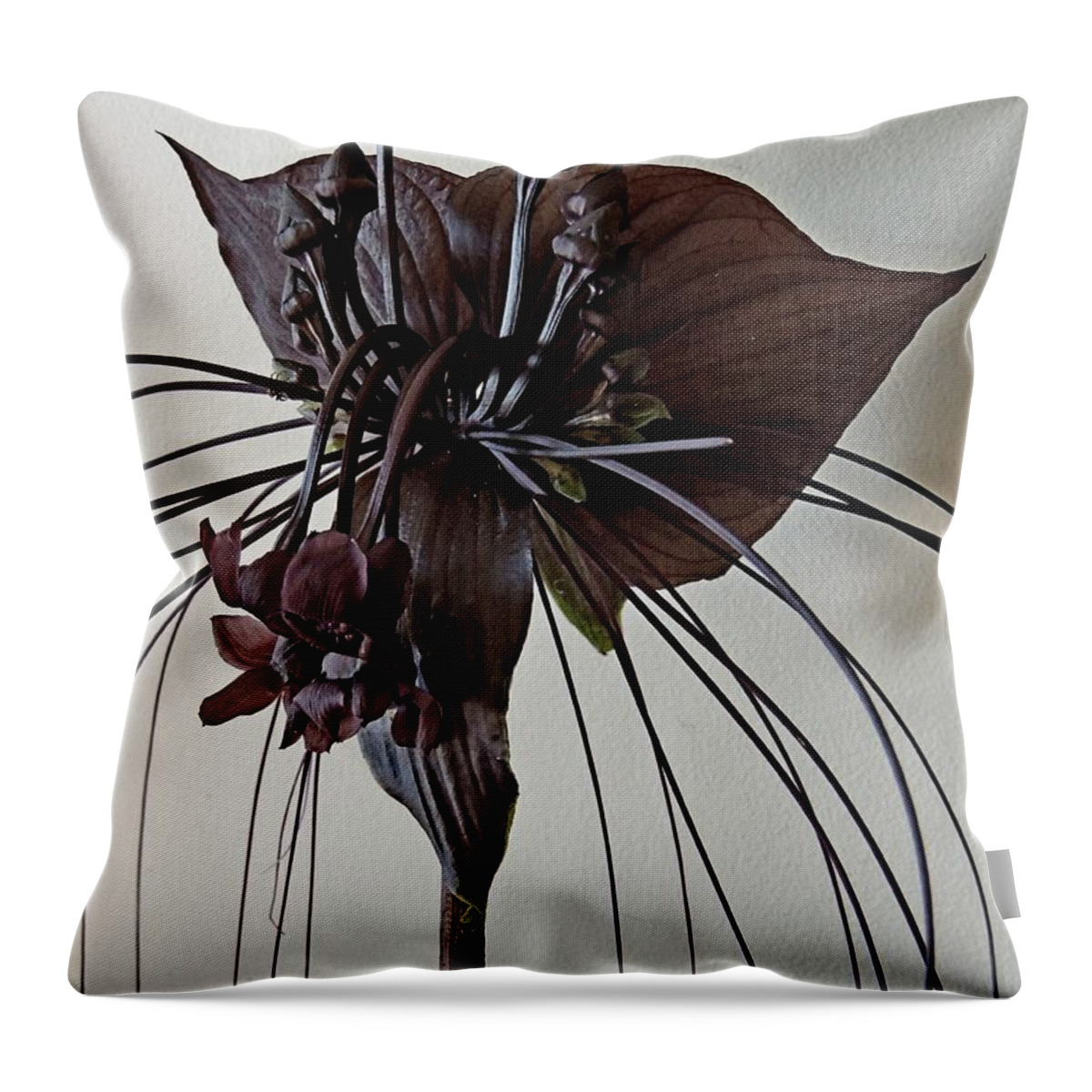This is an image of a decorative pillow with a generally white or cream satin background, tinged slightly with pale gray, especially darker at the top right corner. The pillow, which measures about 12 by 12 inches, features a striking image of a dark floral design that appears to be a black orchid due to its deep and intense hues. The orchid has a complex arrangement of dark purple and dark brown-maroon shades, with delicate green stamens at its center and dark purple fronds and flowers extending outward. The floral design has an intricate pattern that appears to be drawn on the pillow but creates an optical illusion of three-dimensionality, with some elements seemingly emerging from the fabric and hanging down towards the left side. The background of the fabric also carries textures resembling branches, enhancing the depth and complexity of the design. The pillow has a label on the lower right corner, indicating its decorative purpose.